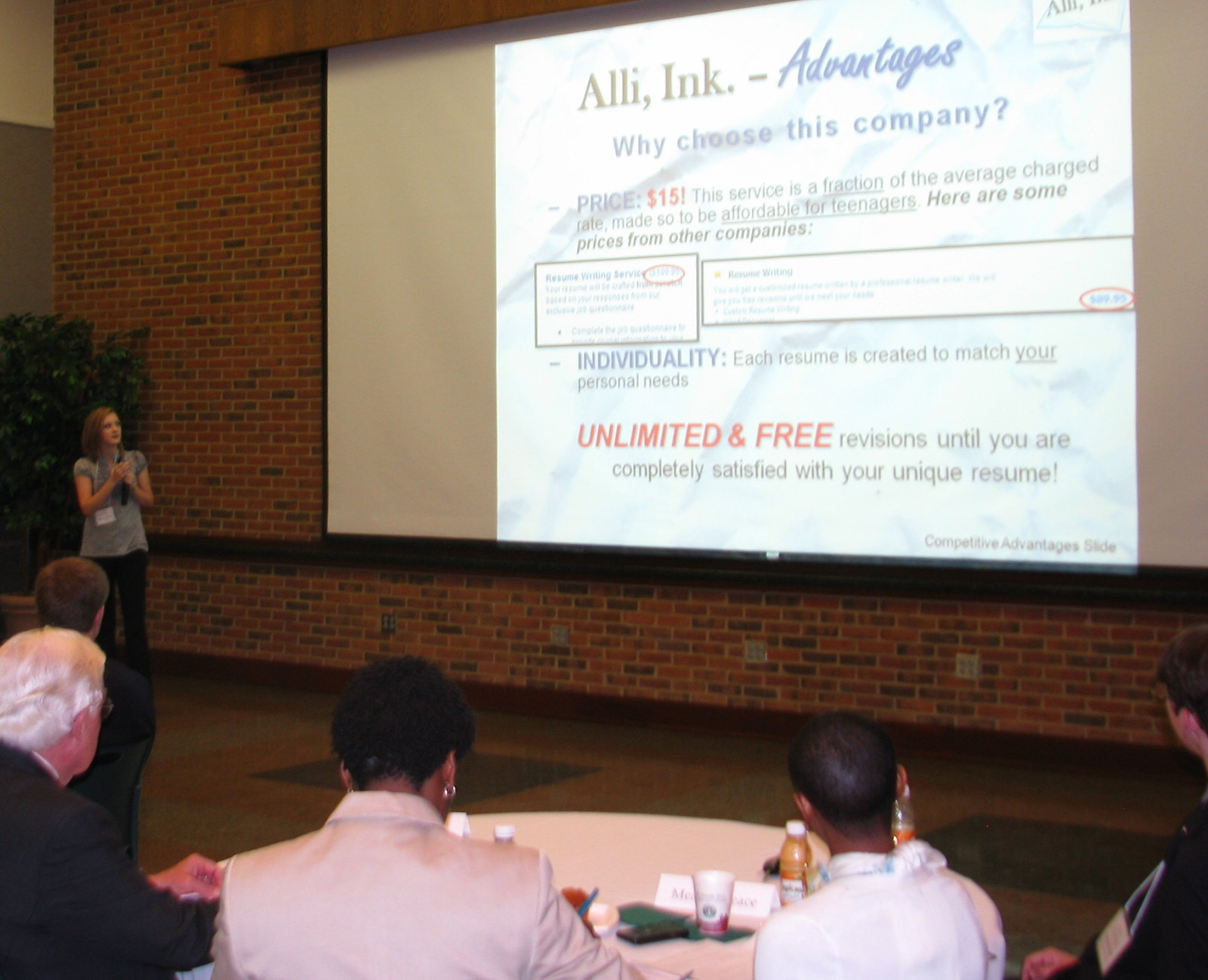The image portrays an indoor company meeting centered around a presentation by a young woman standing on the left side of the room. The woman, who has short reddish-brown hair and is wearing a tan short-sleeved shirt with black pants, holds a microphone with both hands and appears to have a lanyard with a badge near her waist. She is looking up at a large projector screen that displays information about "Ally Inc."

The screen, with a headline reading "Ally Inc. Advantages," presents various points about the company's services. The text includes: "Why choose this company?" followed by "Price $15!" highlighted in red, emphasizing affordability, particularly for teenagers. The slide goes on to state: "This service is a fraction of the average charge rate made to be so affordable for teenagers. Here are some prices from other companies," with two unreadable boxes presumably listing competitor prices. Below these boxes, the text highlights "individuality" by noting, "Each resume is created to match your personal needs." Further down, in red capital letters, it promises "unlimited and free revisions until you are completely satisfied with your unique resume."

In the foreground of the image, another woman with short brownish hair, wearing a gray short-sleeved shirt and black pants, and a lanyard with a badge, is also looking up at the screen. The room features a round table covered with a blush-colored tablecloth, around which five people are seated with their backs to the camera. These attendees include an African-American woman and a boy with short hair on the right, and a Caucasian man with short white hair in a suit on the left, plus another person whose details aren't clear. The scene captures a focused moment of shared learning and information dissemination about Ally Inc.'s resume generation services.